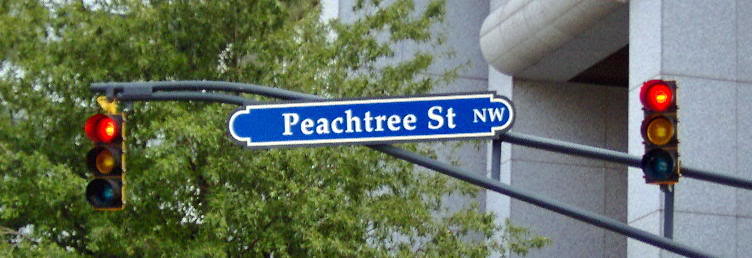This photograph captures a street sign for "Peachtree Street Northwest," which is horizontally rectangular with rounded ends. The sign is royal blue with an internal white border and white lettering. It is mounted on metal rods, which are an army green color, and positioned between two traffic lights, both displaying red signals. In the background, the top of a large, leafy tree is visible, adding a touch of greenery. Beyond the tree stands a substantial corporate building constructed from very pale gray stone, with the entranceway discernible in the frame.